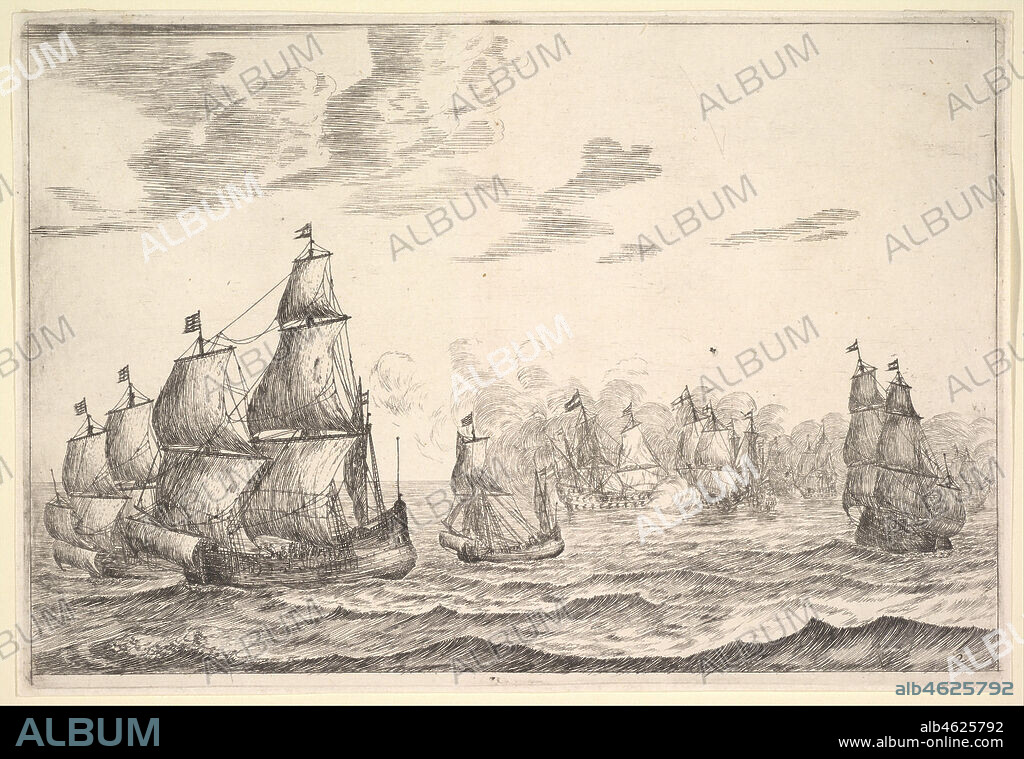The image is a detailed, vintage black-and-white sketch that illustrates a fleet of sailing ships navigating choppy, cresting waves on a stormy sea. The sky is filled with numerous fine-lined clouds stretching across the top half of the image, contributing to the stormy atmosphere. The ships, each equipped with three tall sails raised high on their masts and adorned with flags at the top, vary in size and detail. In the foreground, to the left, lie two prominent vessels, while the center features a smaller, solitary ship. Towards the right, the vessels grow in intricacy, with one ship displaying six large flags on the far right. The scene suggests movement and urgency, possibly indicating an escape or an encounter, as hinted by the smoke trailing behind them. The bottom of the drawing is marked with "ALB 4625792 www.albums-online.com," and a watermark with "ALB" appears in white and gray lettering on the illustration itself.